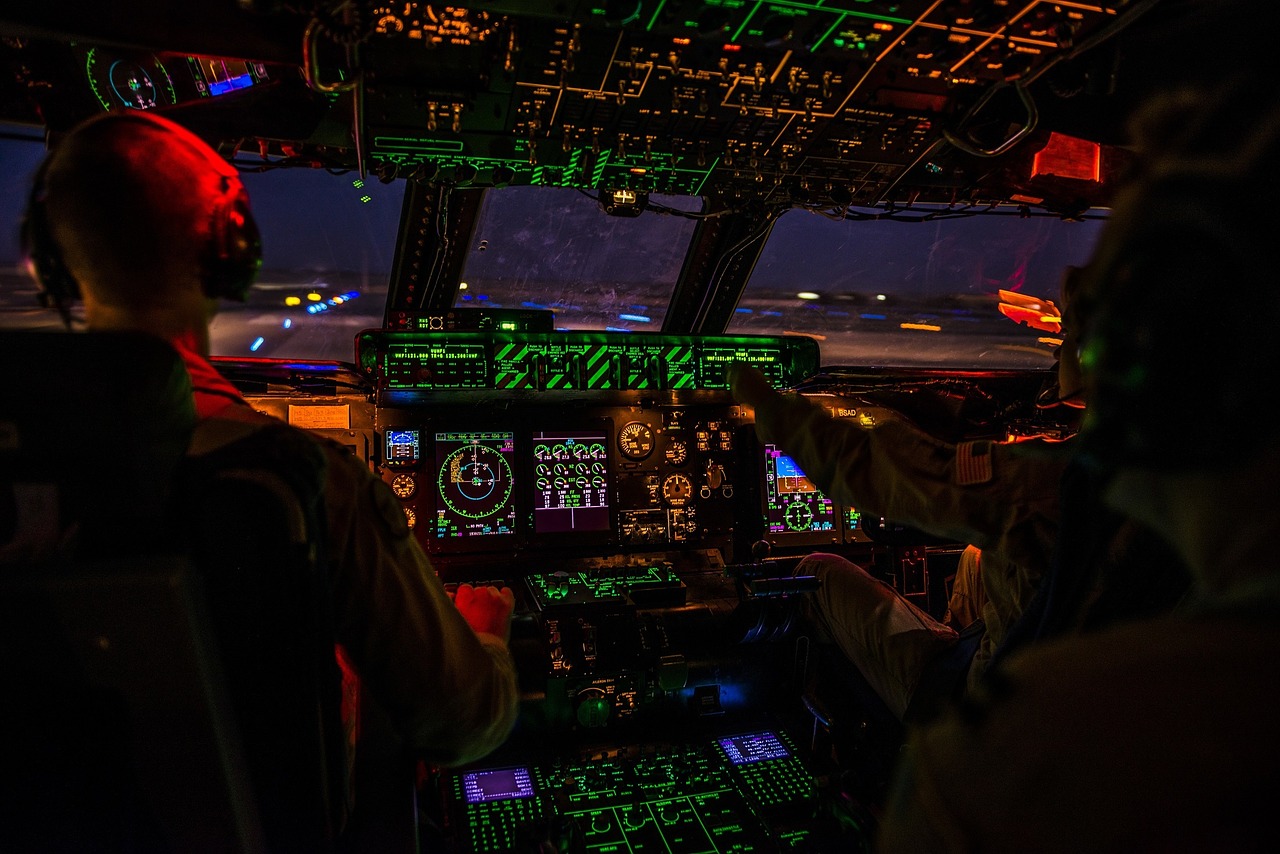In this nighttime photograph of an airplane cockpit taken in vivid color and landscape orientation, two pilots are visible from behind as they focus intently on the dazzling array of instruments before them. The cockpit is illuminated with a mesmerizing array of digital lights and displays, casting a neon glow in hues of vibrant green, pink, orange, and blue. The sheer volume of gauges, dials, and screens speaks to the complexity and high-tech nature of the flight deck. Above the pilots, additional panels brim with illuminated switches and indicators, contributing to the cockpit's futuristic ambiance. Through the front windows of the cockpit, the darkness of night is partially penetrated by a scattering of blurred lights, hinting at a distant cityscape or airport below. The image conveys a sense of intense focus and sophistication, capturing the essence of modern aviation technology against the serene backdrop of the night sky.